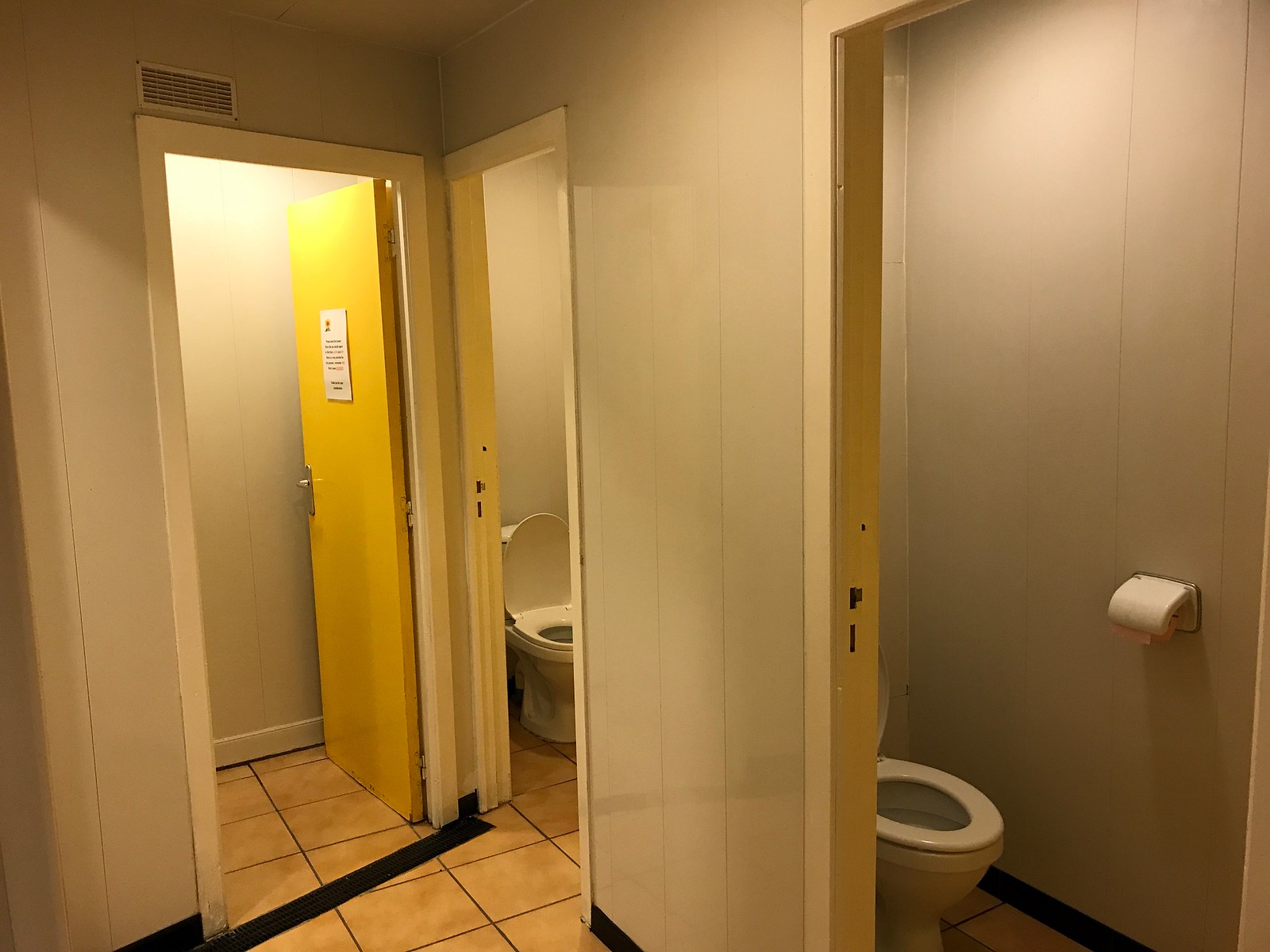This image depicts a bathroom with light beige walls and light brown tiled flooring. On the left side, there is an open yellow door with a silver handle and a sign on it, which provides an opening to another room. The visible portion of the adjoining room has beige-colored walls as well. On the right-hand side, there are two open doors revealing two separate toilet stalls. The back stall contains a white toilet with the lid up, and the stall's back wall holds a roll of light pink toilet paper. Similarly, the front-right stall also features a white toilet with the lid up and a roll of toilet paper on the rear wall. Above the yellow door on the left, there is an air vent visible. The doorframes throughout the bathroom are painted a cream white color, and there are black baseboards along the floor.